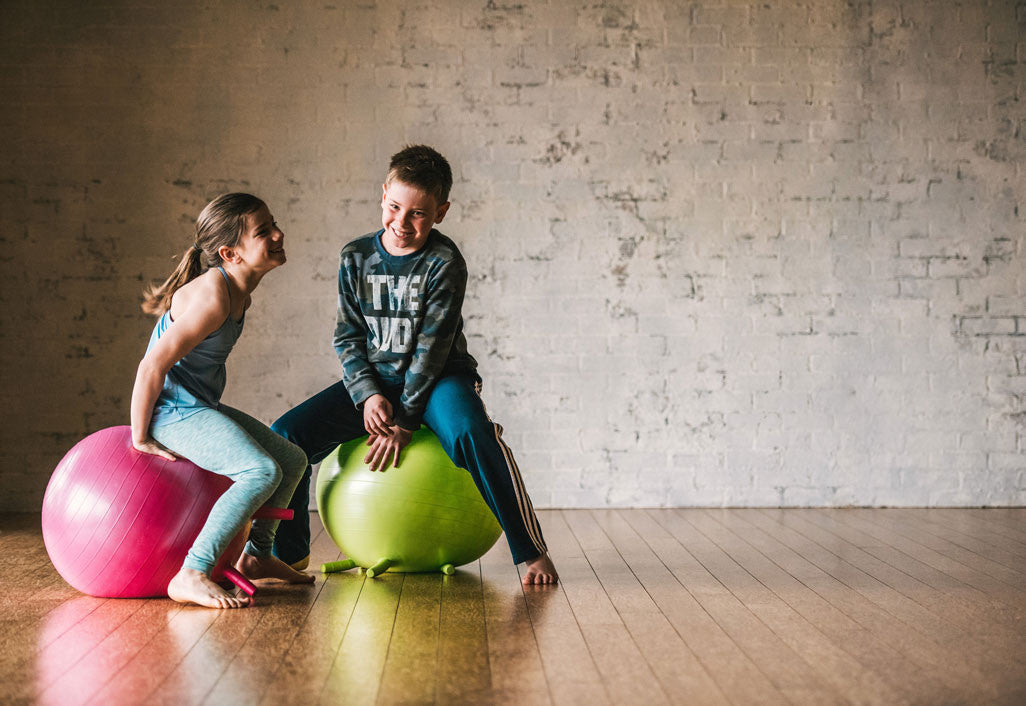In a brightly lit room, two young children are seated on vibrant bouncy balls placed on a light brown wooden plank floor. The background features a white-painted brick wall with faded, chipped sections revealing black specks underneath. On the left, a young girl with brown hair tied back in a ponytail that reaches between her shoulder blades is seated on a pink bouncy ball. She is barefoot and dressed in a light blue tank top and matching light blue pants, with her hands placed underneath her bottom as she balances on the ball. To her right, a young boy is sitting on a green bouncy ball. He has light brown hair styled in short, spiky strands and is smiling brightly. He's wearing a long-sleeved camouflage shirt with the words “The Dude” inscribed across the front and blue workout pants featuring white stripes down the legs. He, too, is barefoot, with his hands placed on the bouncy ball for stability. Both children appear to be having a delightful time, enjoying their playful moment together.